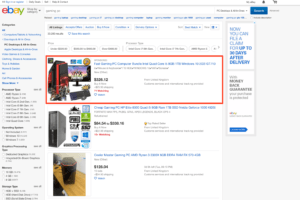The image depicts a screenshot of an older eBay webpage, identifiable by the simple eBay logo, which features a red "e", a blue "B", and a yellow and green "y". The highlighted search term suggests the user was looking for a gaming computer. The cluttered layout of the webpage indicates it's from the late 2000s to early 2010s. The featured gaming PC has a dated, plastic tower with a red and black design and does not include the modern glass side window. The computer bundle appears to come with a monitor and keyboard. Due to the image's size, the price is indiscernible. Below the gaming PC, there is a thinner computer tower and what resembles a coffee mug, adding to the sense of randomness in product display typical of older eBay interfaces.